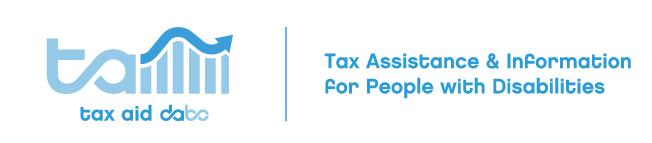The image is a promotional business banner split evenly into two sections by a thin blue line running vertically down the center. The entire background is white, with all elements in blue text. On the left side, the logo features the letters "TA" and incorporates a stylized bar chart with a dark blue curved line and arrow running along the tops of the bars. Below this, it reads "TaxAid.bo" in blue text. On the right side, the banner has the text "Tax Assistance & Information for People with Disabilities," with key terms like "Tax Assistance," "Information," and "Disabilities" capitalized. The ampersand symbol used in the text is creatively designed, resembling an H-shaped symbol. This simplistic yet informative banner serves to promote a tax assistance service specifically for people with disabilities.